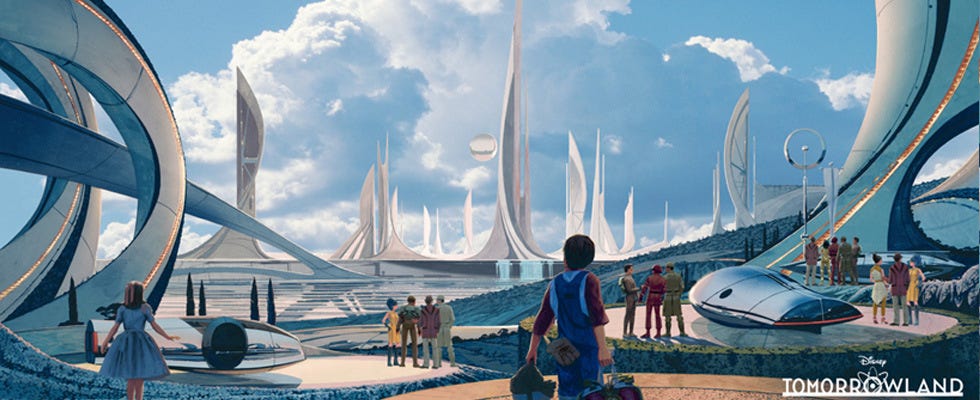This digitally created image, titled "Disney Tomorrowland," is a detailed and mesmerizing portrayal of a futuristic city envisioned by Disney. The title is prominently displayed in a sleek white font, with the "O" in "Tomorrowland" designed with an atomic motif, giving an extra touch of scientific wonder. Dominated by sleek, glassy buildings, the cityscape features shimmering white and silver skyscrapers that spiral and curve elegantly, resembling ice crystals or sailboat sails. The architecture is far from conventional, composed of swirling and curved structures that reach high into the sky, which is a stunning expanse of blue dotted with fluffy white clouds.

Floating in the air are various metallic pods, small spaceship-like vehicles that appear to glide effortlessly without wheels. The streets and open spaces are filled with people dressed in futuristic clothing, some sporting long gloves, boots, fedoras, and ponchos, lending a unique cultural aesthetic to the scene. Among these characters, a notable figure is a little boy in overalls, seemingly from the past, who gazes in awe at the towering structures. A girl in a dress is also observed admiring the skyline, emphasizing the blend of historical innocence and futuristic marvel.

Clusters of people, varying in group size, are scattered throughout, engrossed in conversations and daily activities, contributing to the lively atmosphere of the city. While the landscape is minimal, with a few small trees interspersed among the buildings, the focus on the dense, bustling urban environment underscores the futuristic vision of Tomorrowland.